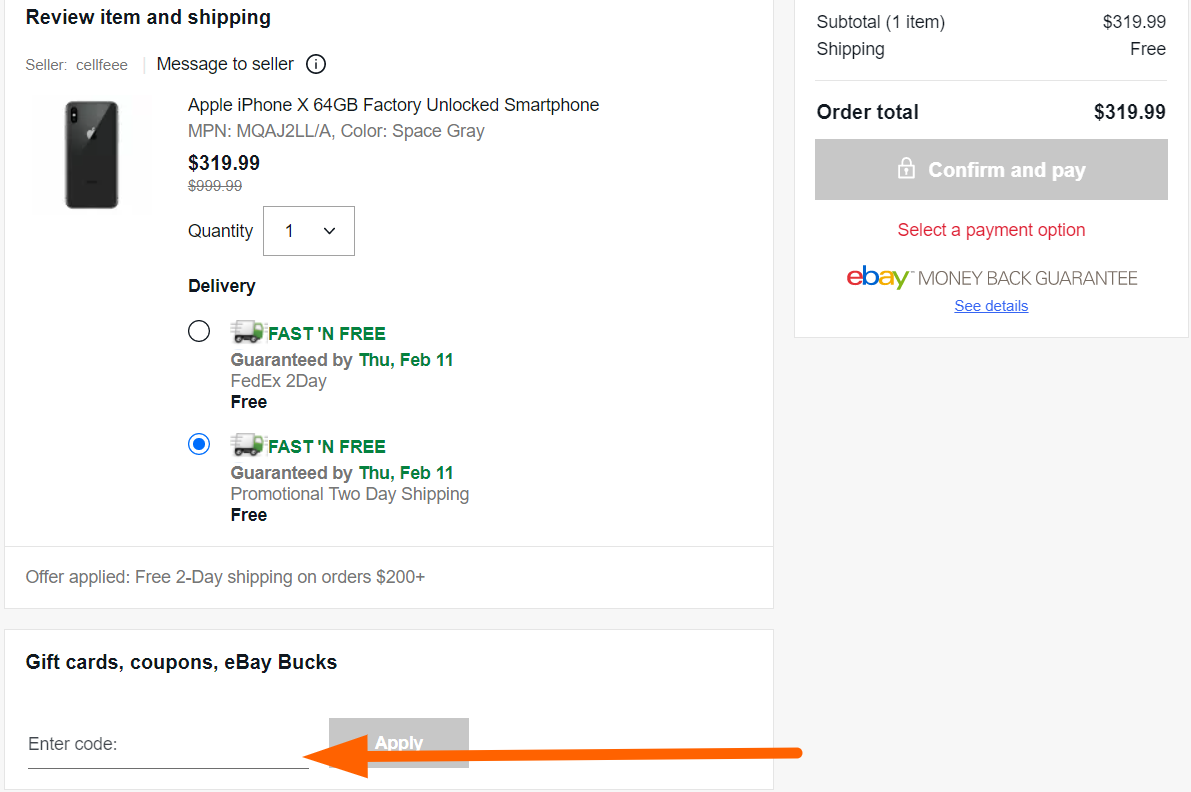This is a photo showcasing an online shopping page for an iPhone X with a 64 GB storage capacity, factory unlocked. The layout is as follows:

1. The left two-thirds of the image has a clean, white background.
2. In the top-left corner, "Review item and shipping" is bolded in black.
3. Directly below, in smaller gray letters, is the description "Seller: selfie."
4. Beneath, there's an image of the back of a black cell phone.
5. To the right of "selfie," there's a prompt saying "Message to seller."
6. Adjacent to this, there's a white circle with a gray border and a gray icon of an eye inside it.
7. Underneath, in black text, it reads "Apple iPhone X 64 GB Factory Unlocked Smartphone."
8. Following this is the model number and color of the phone.
9. Below, you see the price and the quantity selection. There's a gray-bordered square with a "1" inside it.
10. The "Delivery" section offers options - on the left, standard options; to the right, a "Fast and Free" guarantee for delivery by February 11th via FedEx.
11. Under delivery options, a promotional banner reads "Today, Fast and Free February 11th," highlighted in blue.
12. In the bottom left corner, there’s a note: "Applied: Free two-day shipping on orders $200+."
13. Further down, another white rectangle with bolded black text reads "Gift cards, coupons, or eBay bucks."
14. Below is a line indicating "Enter code" with a "Apply" button in gray.
15. An orange arrow points to the "Enter code" section.
16. On the upper right, there's a summary box showing "Subtotal," "Shipping," and "Order Total" with respective prices.
17. Below, a gray tab marked with a white lock icon reads "Confirm and Pay."
18. In red, "Select payment option" is highlighted.
19. At the very bottom, the "eBay Money Back Guarantee" is noted in blue, with a prompt to "See details."

This caption comprehensively details the various elements and sections present in the screenshot of the online shopping page for an iPhone.